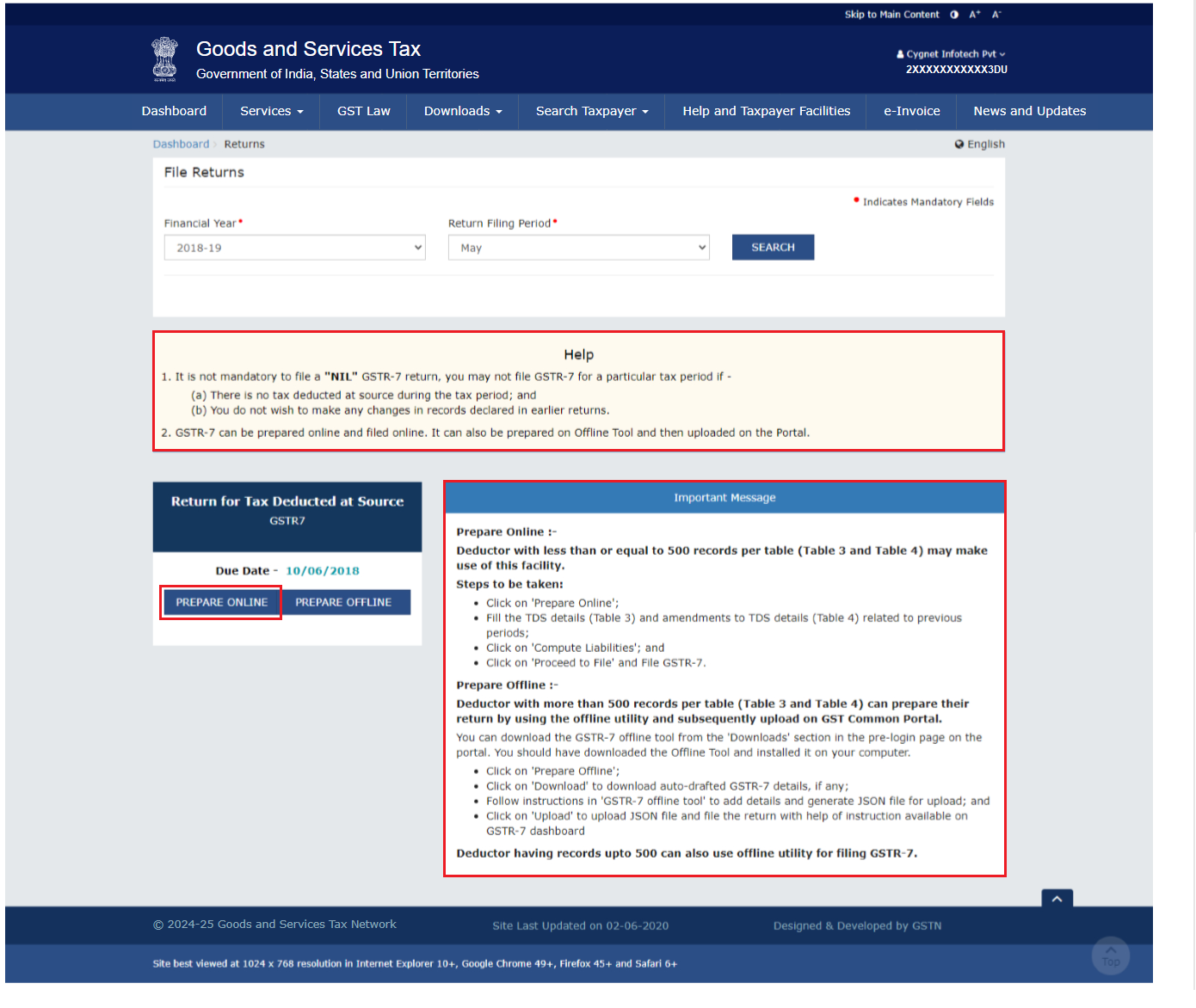Screenshot of the Goods and Services Tax Website:

The image is a screenshot of a web page from the Goods and Services Tax (GST) company. The website features a triple-bar header; the uppermost bar is dark blue, the middle bar is a larger medium blue, and the bottom bar is a smaller grayish blue. 

In the upper left corner, the company name "Goods and Services Tax" is displayed in white text alongside a crown logo, symbolizing the brand. On the upper right, there are navigation links including "Skip to main content" and other site shortcuts.

The grayish blue bar below displays a horizontal menu with options from left to right: "Dashboard," "Services" (with a dropdown menu), "GST Law," "Downloads" (with a dropdown menu), "Search Taxpayer" (with a dropdown menu), "Help and Taxpayer Facilities," "New Return Trial" (with a dropdown menu), and "E-Invoice."

The main content area shows that the user is on the "Dashboard" for tax returns. This section includes an option to file returns with a fiscal year dropdown menu (selecting 2018-19) and a return filing period dropdown menu for selecting the month. Adjacent to these dropdowns is a search button.

Below this, the screen prompts with a line that says, "If you need help," followed by directions and a link to tax deadlines and resources. The bottom right section highlights an important message area that provides critical updates regarding tax filings.